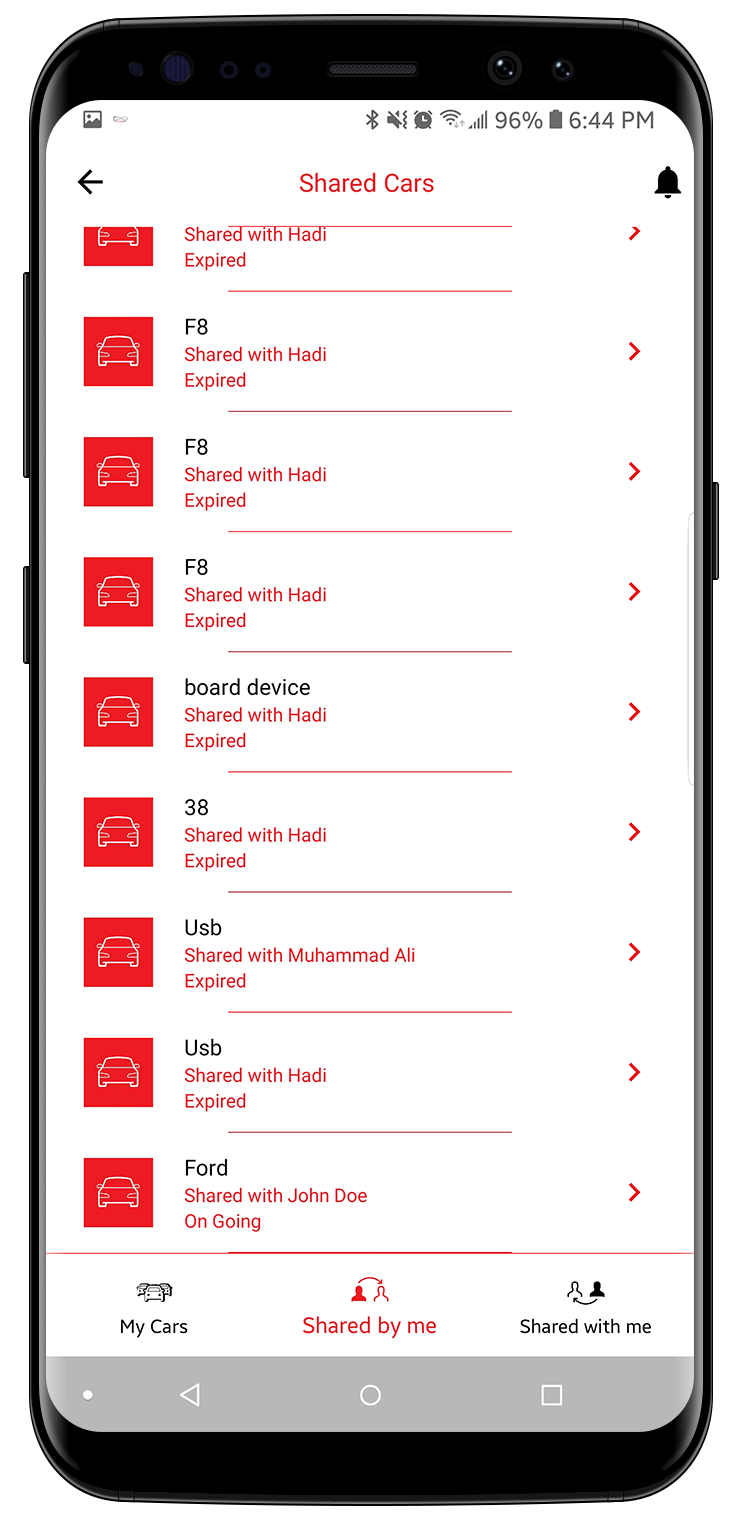This image appears to be a detailed mock-up of a generic smartphone. The phone's display shows a reflection on the glass, accentuated by side buttons and a visible frame, although it notably lacks an iconic bottom button typical of an iPhone. The upper section of the screen is populated with standard icons: a photo icon on the left, and on the right are indicators for Bluetooth, speaker off, an alarm, Wi-Fi signal, mobile network strength showing full bars, a 96% battery indicator, and the time, 6:44 PM.

Central to the image is an inset panel, possibly simulating a screenshot. Dominating the screen is the text "Shared Cars" in red, with several entries listed below. Each entry features a red car icon on the left and a red arrow on the right. Among the entries, text elements like "Shared with Hottie" and "Expired" are prominently in red, while identifiers like "F8," "Board Device," "38," "USB," and "Ford" are in black.

At the bottom of the screen, navigation items are listed in separate sections labeled "My Cars," "Shared by Me," and "Shared with Me," though the exact order may differ. The overall design emphasizes connectivity and management of shared vehicles, likely intended for a transportation or car-sharing app interface.